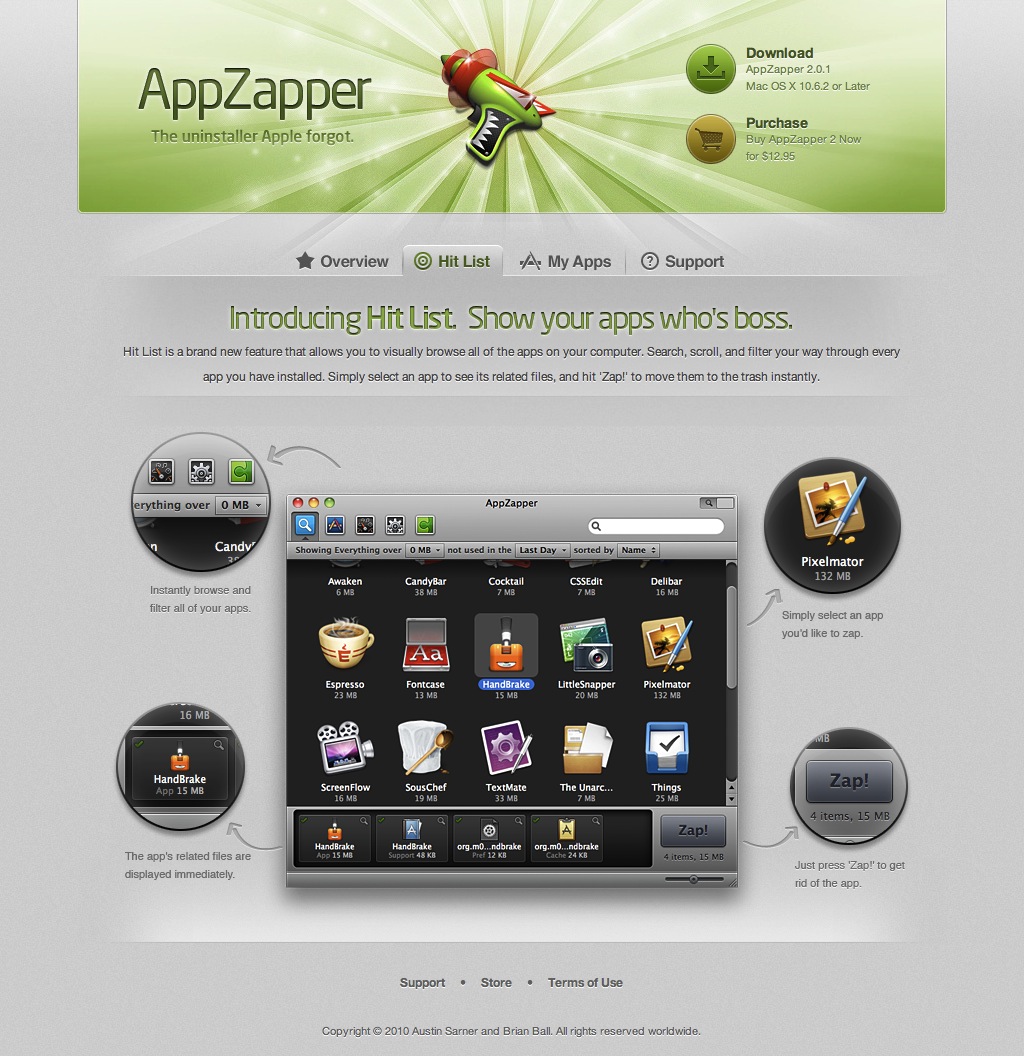The image depicts a detailed advertisement for AdZapper, styled as a website or poster. At the top, the AdZapper logo, characterized by green coloring with white stripes, stands prominently. The tagline "App Zapper: The uninstaller Apple forgot" is displayed in a green box. Central to the image is a visually striking, toy-like futuristic zap gun in green and red, symbolizing the app’s functionality. To the right, the options to "Download" or "Purchase" the app are highlighted.

Just below these primary elements, tabs labeled “Overview,” “Hit List,” “My Apps,” and “Support” are presented, with the "Hit List" tab selected. The central screenshot within the advertisement emphasizes the "Hit List" feature, showcasing how it allows users to browse through their apps efficiently with the slogan "Show your apps who's boss" in green text. Below, detailed descriptions explain that Hit List enables users to visually browse, search, scroll, and filter apps. Users can select an app, view related files, and instantly remove them by pressing "Zap."

Supporting visuals on each corner of this central screenshot provide quick tips: "Instantly browse and filter all your apps," "The app's related files are displayed immediately," "Simply select an app you'd like to zap," and "Just press zap to get rid of the app." Additional navigation options, such as "Support," "Store," "Terms of Use," and "Copyright Information," are found at the bottom of the web page preview, completing the comprehensive layout of the AdZapper advertisement. The color scheme throughout the ad is multicolored, mainly utilizing green and black, with vivid app icons enhancing the central visual appeal.